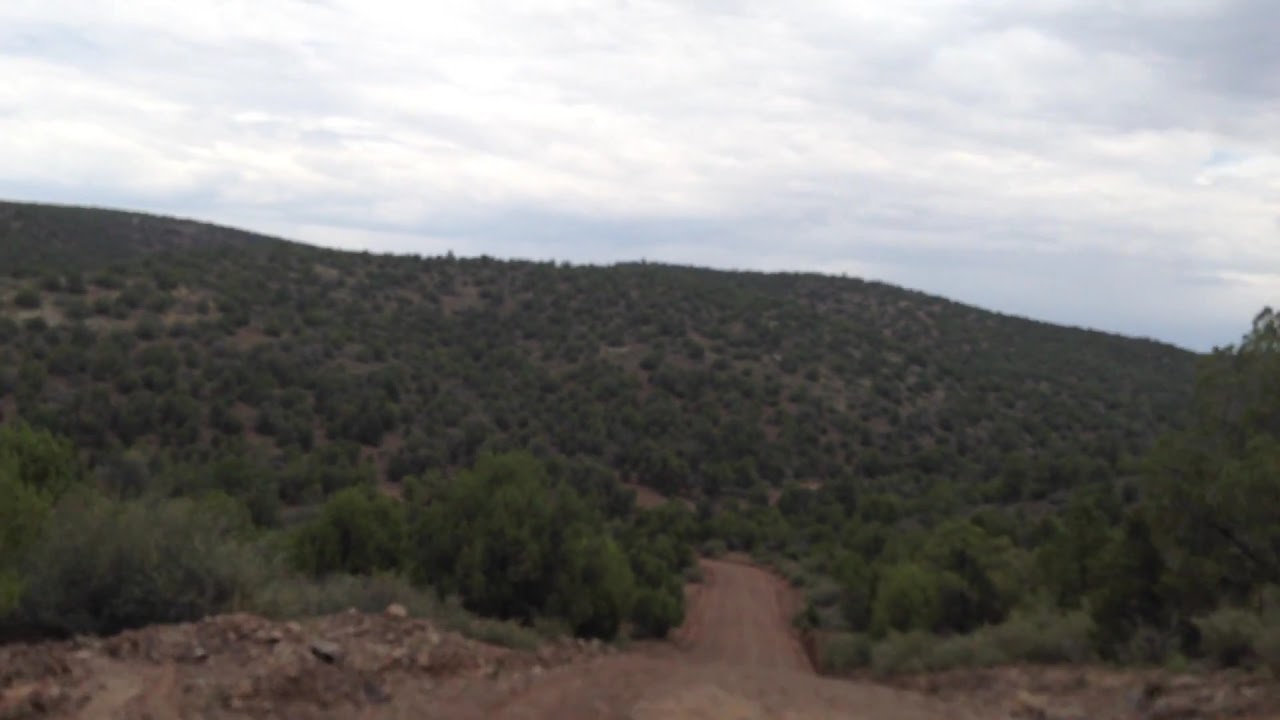The photograph showcases a sprawling natural scene dominated by a winding dirt road and rolling foothills. Starting at the bottom center, a red dirt road, flanked by rocks on its left side, travels upwards before vanishing behind the hills, likely turning left. The landscape is covered with short shrubs, bushes, and patches of colorful greenery that extend across the entire foreground and middle ground, suggesting a serene yet rugged wilderness. The background reveals a continuous expanse of green hills interspersed with trees and other vegetation. Above, the sky is overcast and filled with dense white and gray clouds, devoid of any visible blue sky or sunlight. The image, with no visible man-made structures or people, encapsulates the raw beauty of a secluded outdoor environment, likely captured in the middle of the day.